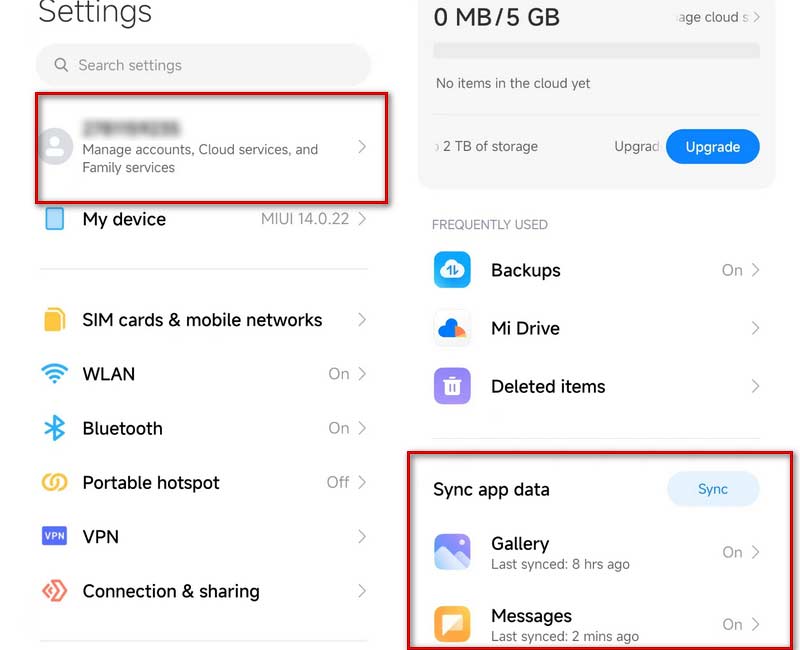The image consists of two smartphone screens with detailed settings and cloud service information.

**Left Screen:**
- **Background:** White
- **Heading:** "Settings"
- **Top section (partially blocked):** Unspecified content
- **Search bar:** "Search settings"
- **Sections:** 
  - "Manage accounts"
  - "Cloud service"
  - "Family services"
- **Subsections:**
  - "My device"
  - "SIM cards and mobile networks"
  - Connectivity options such as:
    - "Bluetooth" (ON)
    - "Portable hotspot" (OFF)
    - "VPN"
    - "Connections and sharing"

**Right Screen:**
- **Cloud storage details:**
  - "0 MB of 5 GB used"
  - "Cloud" section noting "no items in the cloud yet"
  - "Upgrade storage" option with a blue button labeled "2 TB of storage"
  - Options under cloud services:
    - "Backups"
    - "My Drive" (or "Mi Drive")
    - "Deleted items"
- **Highlighted section (red box):** "Sync app data"
  - Blue button with green font labeled "Sync"
- **Sync status:**
  - "Gallery" (last synced 8 hours ago)
  - "Messages" (last synced 2 minutes ago)

**Color Scheme:**
- Dominant colors include purple, blue, orange, red, white, black, gray, and possibly some intermediate hues like yellow-green and orange-yellow.

This detailed description encapsulates the key elements and functions displayed across the two smartphone screens, highlighting their respective sections and sync statuses.